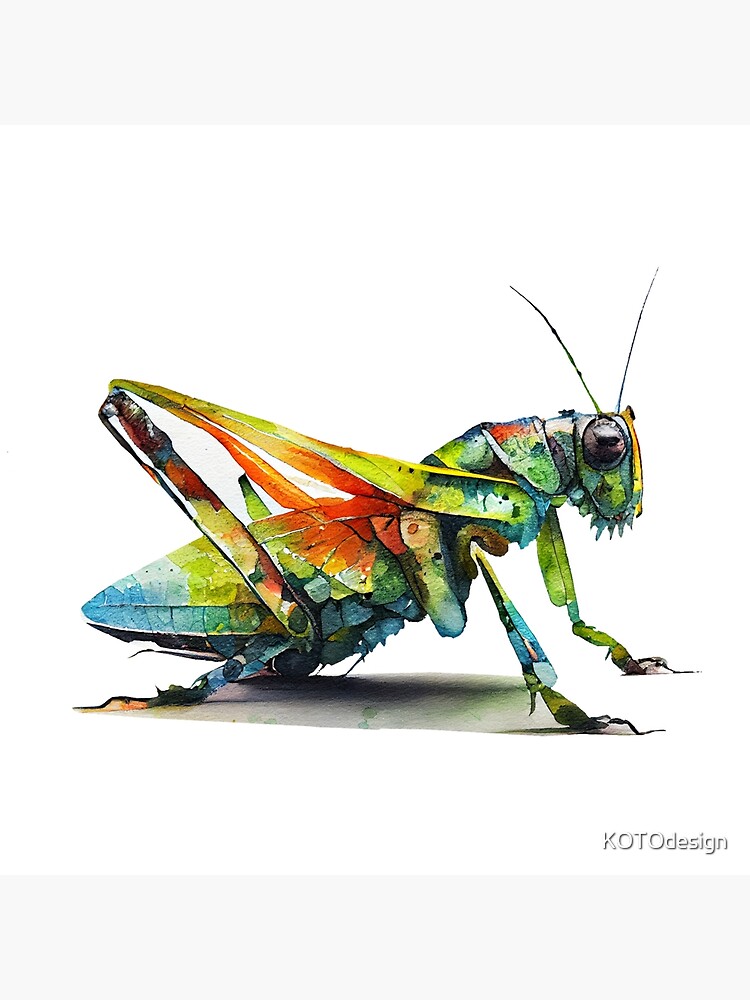This vibrant artwork features a grasshopper rendered in a watercolor-like style on a pristine white canvas. The grasshopper is depicted from a side view with its head facing the right and its tail to the left, positioned on the ground with its back legs bent in a relaxed posture. The head showcases a light blue hue complemented by dark black eyes and green and blue antennae. The grasshopper's body is a stunning mix of colors, including green, blue, orange, yellow, red, and black, intricately blending to form its shape. The wings protruding toward the legs are primarily yellow with hints of blue and orange. The legs exhibit a combination of blue, green, brown, and red, creating an almost metallic appearance. Subtle shadows beneath the grasshopper add depth to the piece. The artwork, signed "Koto design" in the bottom right corner, completes this eye-catching composition.